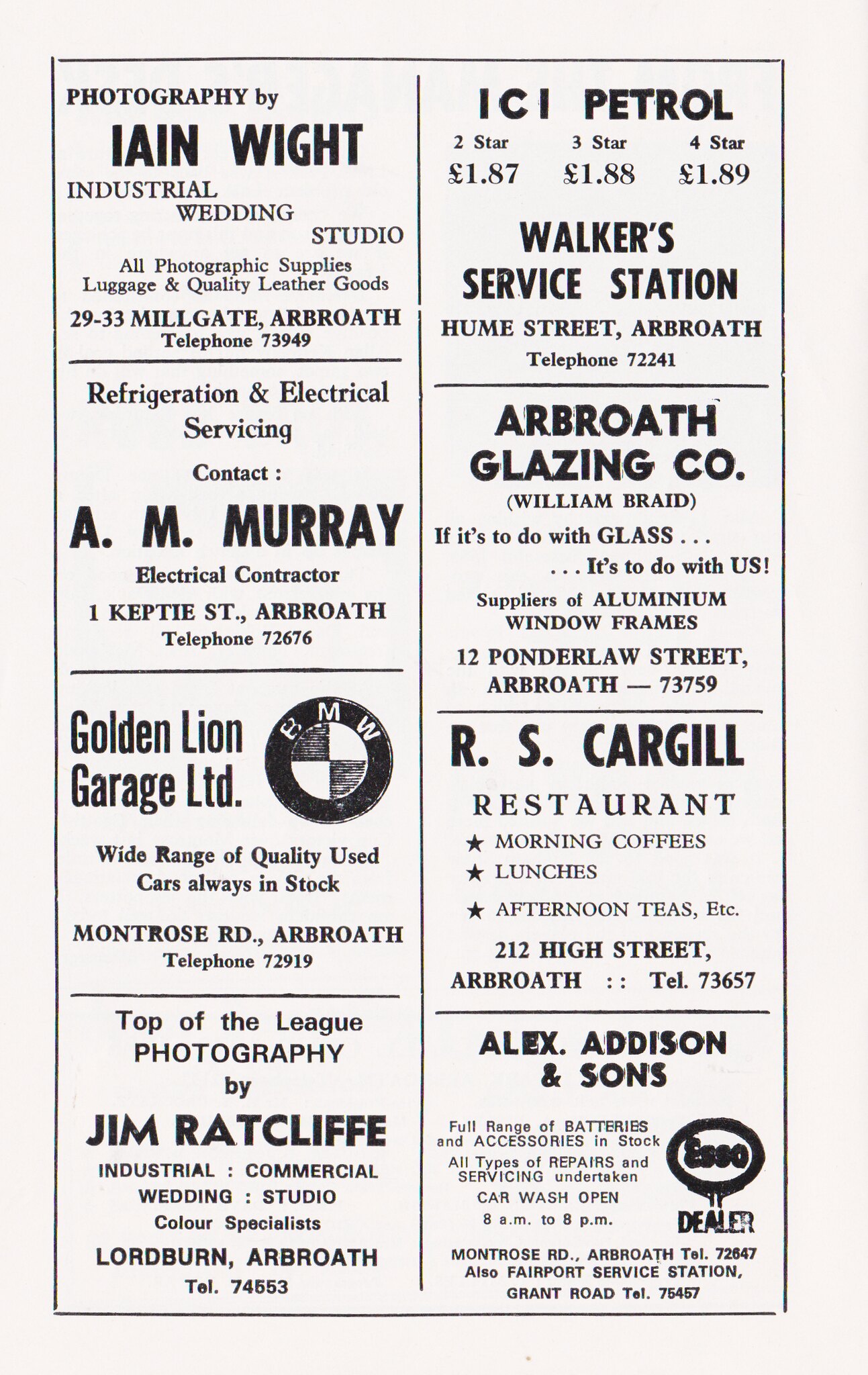The image features a vintage page from a magazine or newspaper densely packed with advertisements for local businesses in Arbroath. The layout consists of eight boxes, four on each side. Starting from the top left, the first ad showcases "Photography by Iainwigh" of the Industrial Wedding Studio located at 29-33 Milligate, available at Telephone 73949. Below that, there's another box for "Refrigeration and Electrical Servicing" which prompts readers to contact A.M. Murray, Electrical Contractor, at Kepty Street. Further down, the "Golden Lion Garage Limited" advert highlights a dealer with a white BMW logo, offering a selection of used cars in various colors, based on Montrose Road with Telephone 72919.

On the right side, from top to bottom, the first box promotes "ICI Petrol" with 2, 3, and 4-star fuel options, available at Walker Service Station on Hume Street, Telephone 72241. Next, the "Arbroath Glazing Company" run by William Brayne claims, "If it's to do with glass, it's to do with us," specializing in aluminum window frames at 12 Ponder Law Street, Telephone 73759. Below that, the "R.S. Cargill Restaurant" is advertised for its morning coffees, lunches, and afternoon teas, at 212 High Street, Telephone 73657. The last advert on this side is for "Alex Addison and Sons," offering a full range of batteries, accessories, repairs, and servicing, with a car wash open from 8 AM to 8 PM, located on Montrose Road, Telephone 72647. Additionally, they mention "Fairport Service Station" on Grant Road, Telephone 75457, where they are an ESSO dealer.

In summary, the image is an old print ad page primarily marketing various local Arbroath businesses, including photography services, automotive services and sales, fuel stations, glazing and glassworks, and dining options, complete with detailed contact information and locations.